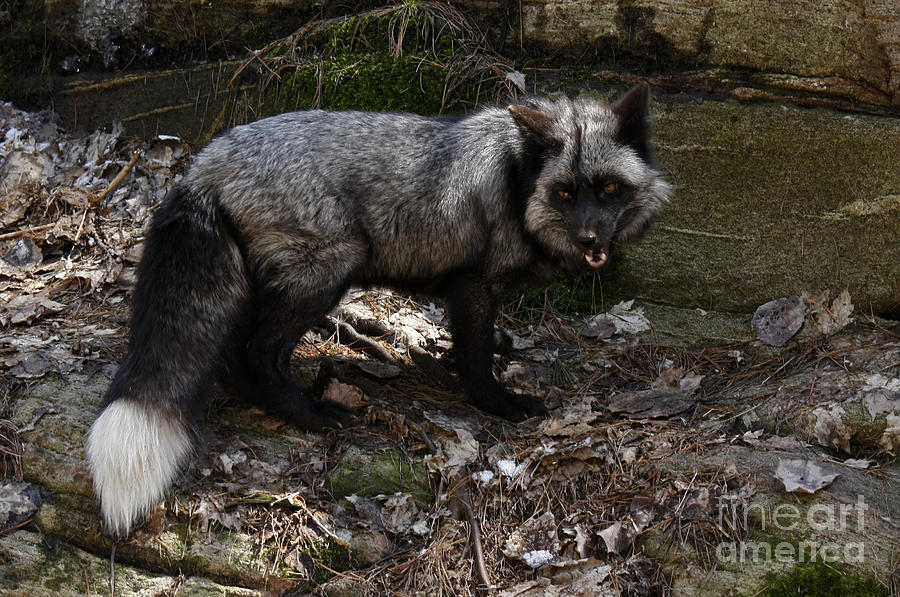This detailed photograph captures a striking silver fox standing amid a wooded area filled with leaves, twigs, and pine needles. The fox is facing to the right, yet its head is turned towards the camera, offering a direct gaze with reddish-brown eyes. Its mouth is open, revealing the bottom teeth. The fox's coat features a beautiful, thick black tail tipped with white and a speckled silver-gray fur, giving it a salt-and-pepper appearance. Its ears are primarily black, and its face includes black markings around the eyes, a black nose, and white cheek regions.

The fox's legs and belly are also black, contrasting with the silver-gray of its body. In the background, one can observe a wooded area with broken branches, twigs, and rocks covered with moss. Roots run through the area, adding to the natural scenery. The overall tone of the image is somewhat muted, providing a gray, subdued color palette that enhances the fox's unique coloration.

Adding to the composition, the bottom right corner of the image features the watermark "Fine Art America," where "Art in America" appears in bolder letters compared to "fine." The sunlight filtering into the scene hints at a likely morning setting.